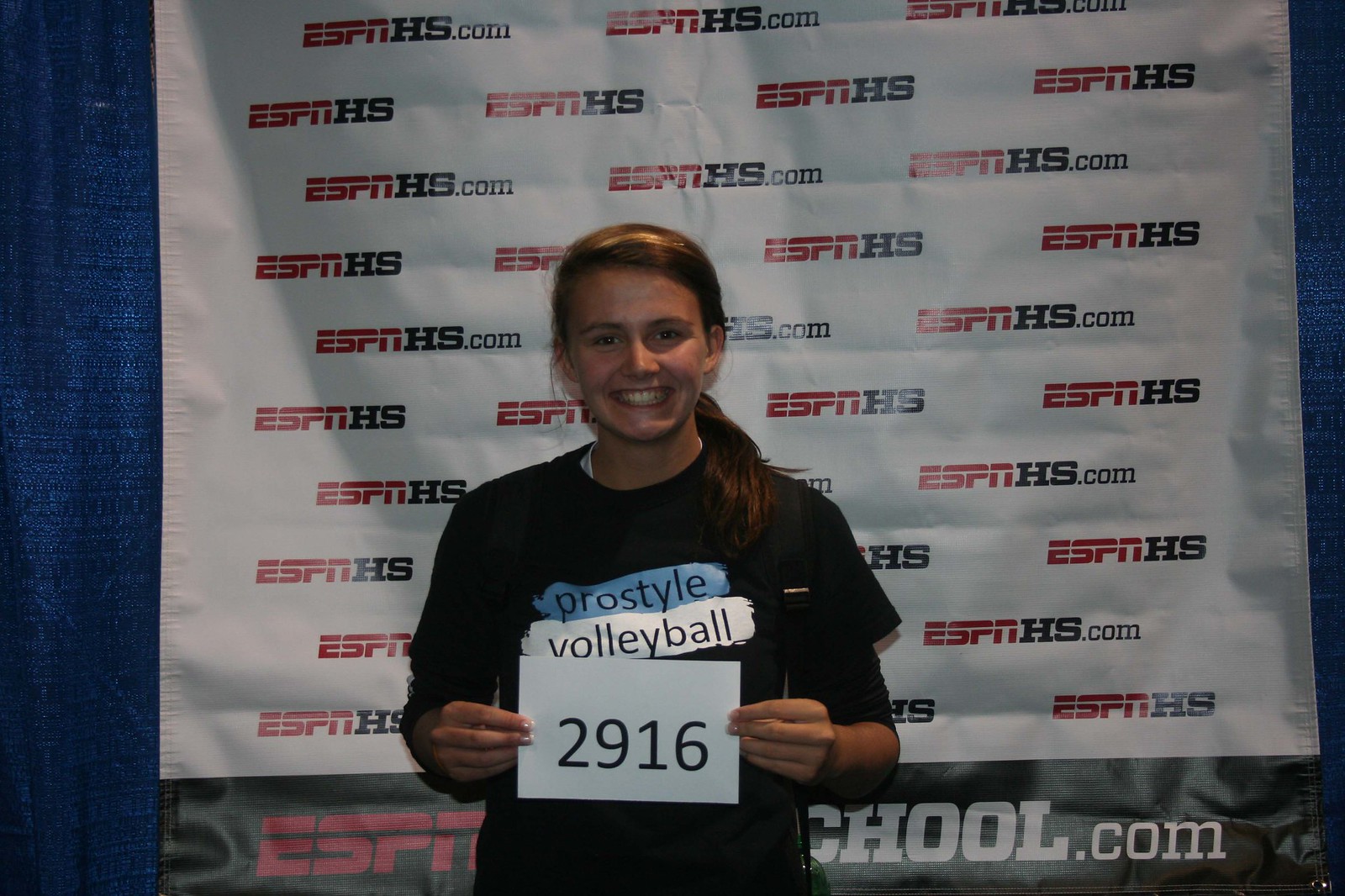This horizontal rectangular photograph features a young woman, likely a high school volleyball player aged around 16 or 17, standing centrally against a backdrop. The backdrop prominently displays the repeated phrase "ESPN HS.com" with "ESPN" transitioning from orange to red, "HS" in black, and the "dot-com" in a slightly lighter black. The banner is white and partially extends on the lower left side where a blue curtain starts. 

The young woman is smiling at the camera, wearing a black t-shirt that reads "ProStyle Volleyball." The text 'ProStyle' is set against a blue background, while 'Volleyball' is displayed within a white stripe, though some earlier descriptions may have misread the shirt details. She holds a white card displaying the number "2916" with the word "volleyball" written above it, which is likely her player number for the team. The photograph emphasizes the volleyball player centered in the image, her black t-shirt with blue and white accents, and the ESPN branding in the backdrop. The primary colors in the image are black, white, red, and blue, creating a sharp, vivid contrast.